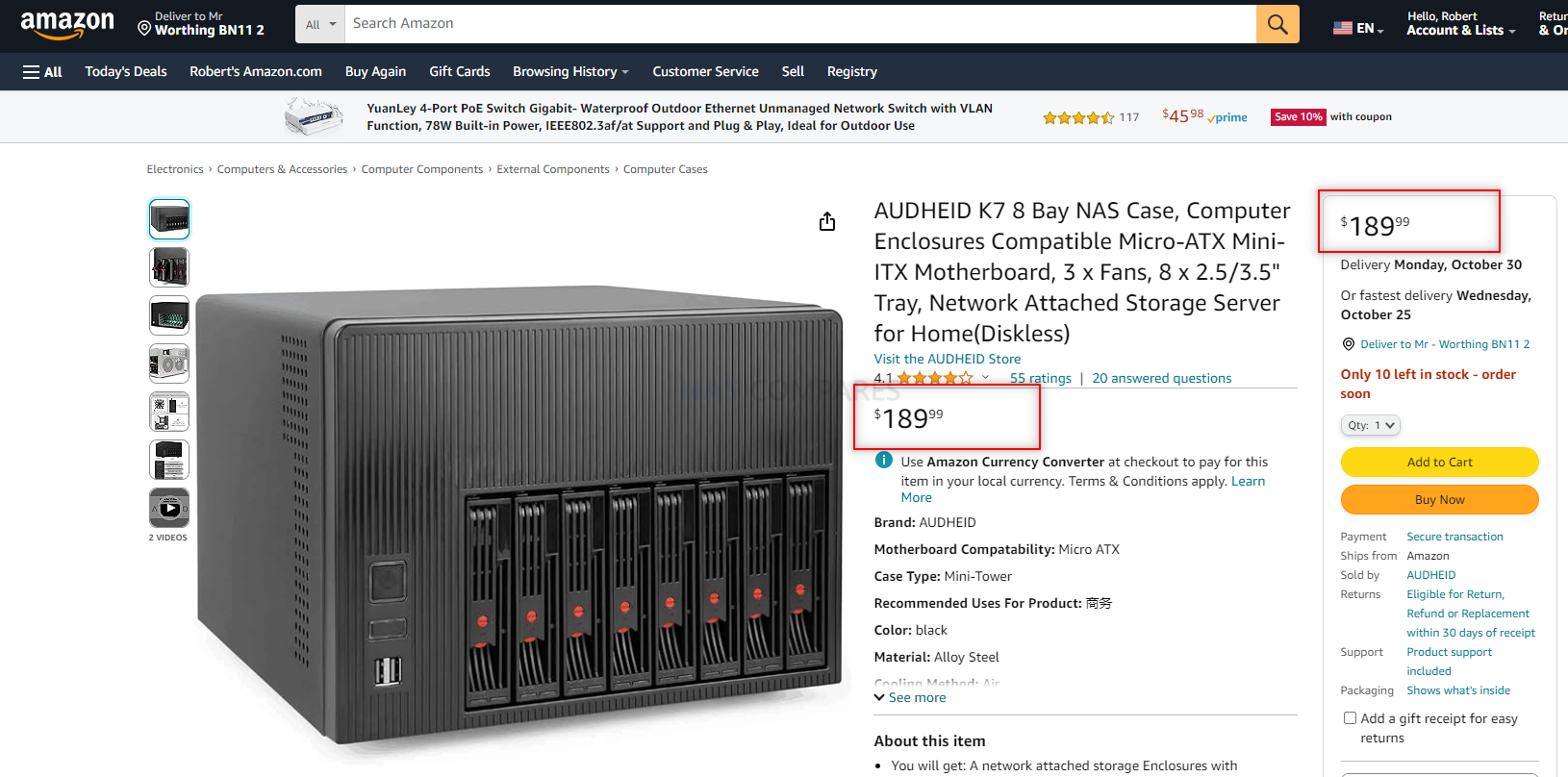The image depicts an Amazon.com shopping page featuring a product listing for a black storage server. At the top of the page, the Amazon logo is prominently displayed with the company name written in white letters accompanied by an orange arrow. Just beneath the logo is a search box with the placeholder text "Search Amazon," and a magnifying glass icon is located next to it. To the right, a small American flag icon next to the letters "EN" indicates that the page is displayed in English.

The central focus of the page is a large image of the black storage server. The price, highlighted with a red box, is prominently shown as $189.99 in bold black text. Below the price, delivery options are stated: standard delivery by Monday, October 30th, or the fastest delivery by Wednesday, October 25th, also in black text. A warning in red text indicates that only 10 units are left in stock, urging customers to order soon.

To the right of the product image, there is a quantity selection box currently set to "Quantity: 1" with a down arrow for adjusting the amount. Directly below this, a yellow rectangular button with black writing invites users to "Add to Cart," and beneath that, an orange rectangular button with black text offers the option to "Buy Now."

The section titled "About this item" starts to describe the product features, noting that the user will receive network-attached storage enclosures.